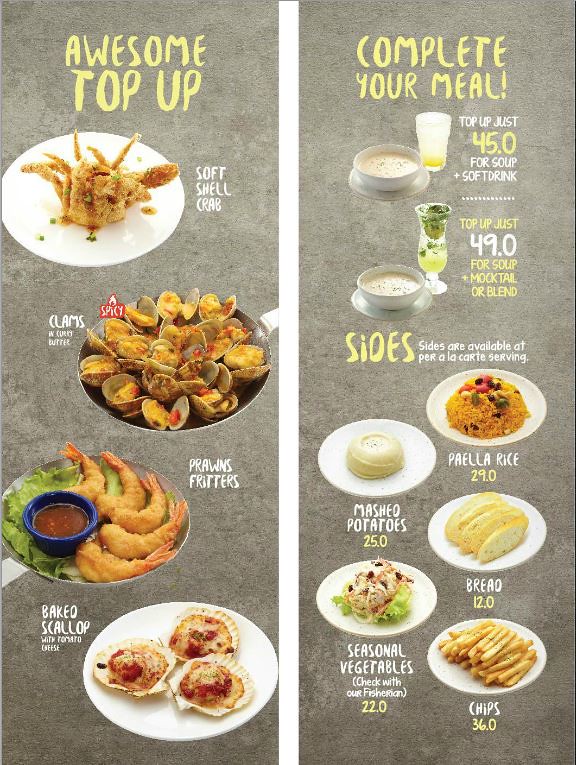This image displays a menu divided into two columns with a gray background. The left column, titled "Awesome Top-Up" in yellow, showcases four mouthwatering dishes: Softshell Crab highlighted with a white plate icon, Clams Spicy denoted by a pan image, Prawns Fritters shown with prawns on a bed of lettuce, and Baked Scallops with Tomato Cheese indicated by a plate graphic. The right column, crowned with "Complete Your Meal" in yellow, offers enticing drink and side options. It features a promotion for a bowl of soup and a soft drink at just $45, and another for a soup and mocktail or blend at $49. Additionally, there are a la carte side dishes, each with a corresponding image: Paella Rice ($29), Mashed Potatoes ($25), Bread ($12), Seasonal Vegetables (price varies, check with the Fisherman, $22), and Chips ($36).